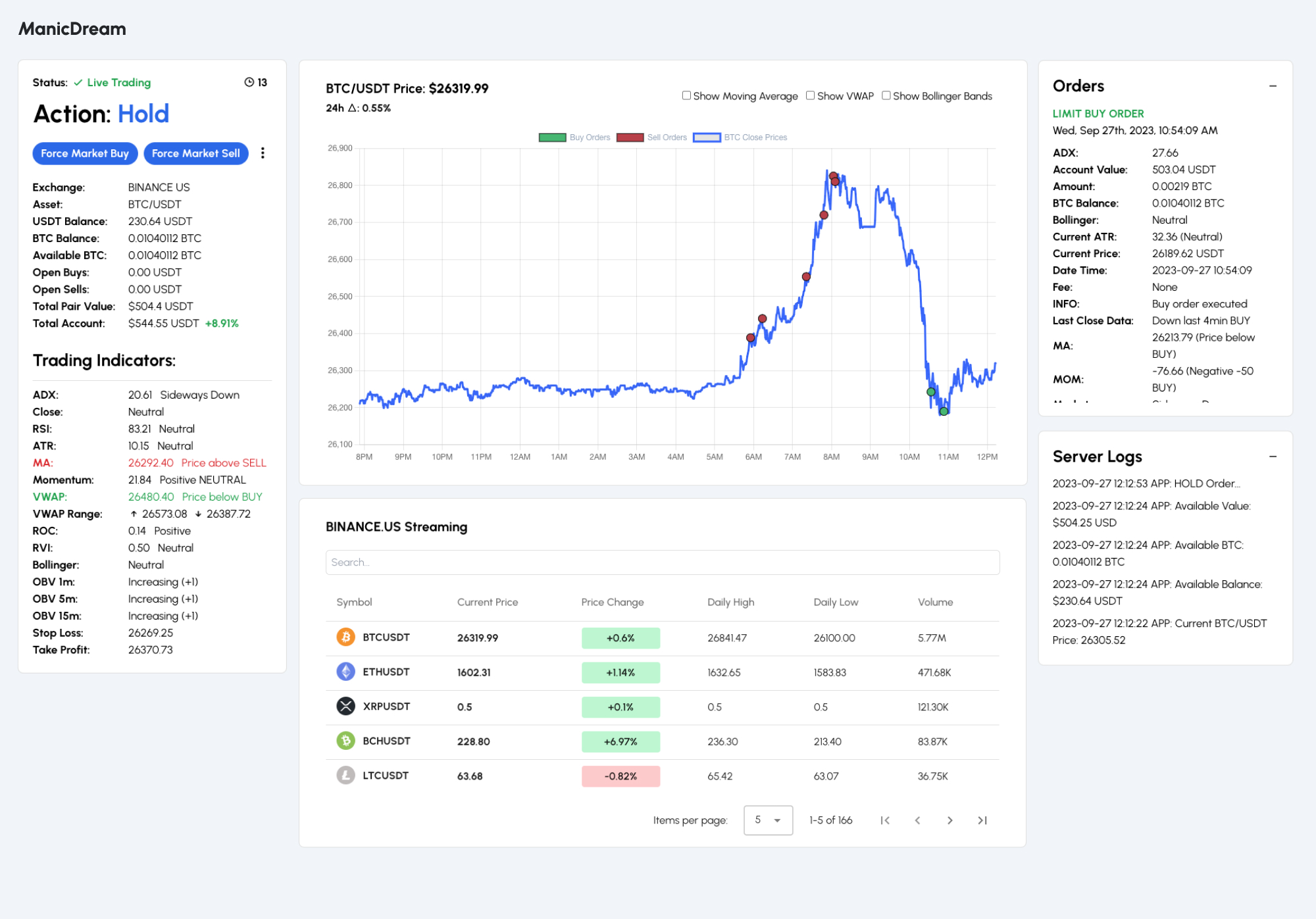The image showcases a web page from "Manic Dream," with the site's title prominently displayed in the upper left-hand corner. On the left side of the page, there is a box labeled "Action Hold," providing various pieces of information possibly related to stock trading. This section includes options to buy and sell stocks, with interactive blue buttons to execute these actions. It also features trading indicators and statistics for different stocks.

At the top of the page, a larger white box displays the current price for the BTC/USDT pair, accompanied by a line graph. The graph begins with a flat trend, then rises sharply to a peak before declining steadily, followed by a minor rebound. The page also mentions "Finance U.S. Streaming," with various statistics beneath this heading. Some of these stats are highlighted in green, while one is highlighted in pink, presumably indicating key financial metrics or alerts.

On the right side of the page, a section titled "Orders" details limit buy orders, including an entry dated Wednesday, September 27th. Below this, a smaller box labeled "Server Logs" provides additional technical information. Overall, the web page appears to track and display real-time stock activity and related data.